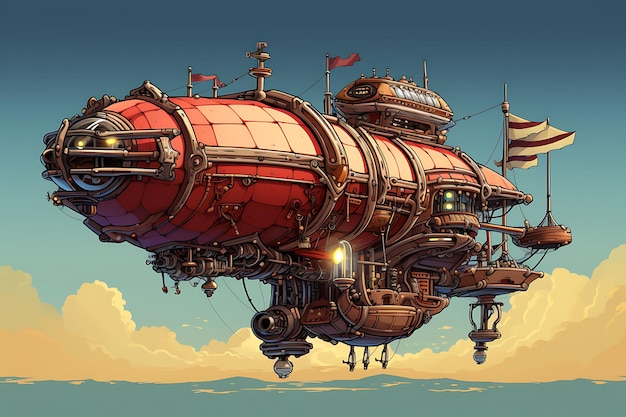The image is a detailed graphical cartoon of a massive, intricately designed flying airship or zeppelin, which resembles a castle and could potentially be a warship. The airship is floating majestically in the sky above a vast, blue, wavy sea. Above the waves, the skies are filled with creamy white, fluffy clouds and transitions into a clear, darker blue as you look higher. The airship itself boasts a reddish and beige color palette, with some purple hues at the bottom. It is adorned with various flags: a prominent red flag hoisting at the top and white and black striped flags hanging beneath. Adding to its elaborate appearance, the airship has lights switched on; some appearing as golden red lights, and others situated towards its sides, resembling eyes. The entire scene is set in a vibrant outdoor setting, enhancing the surreal and fantastical nature of the flying castle-like ship.